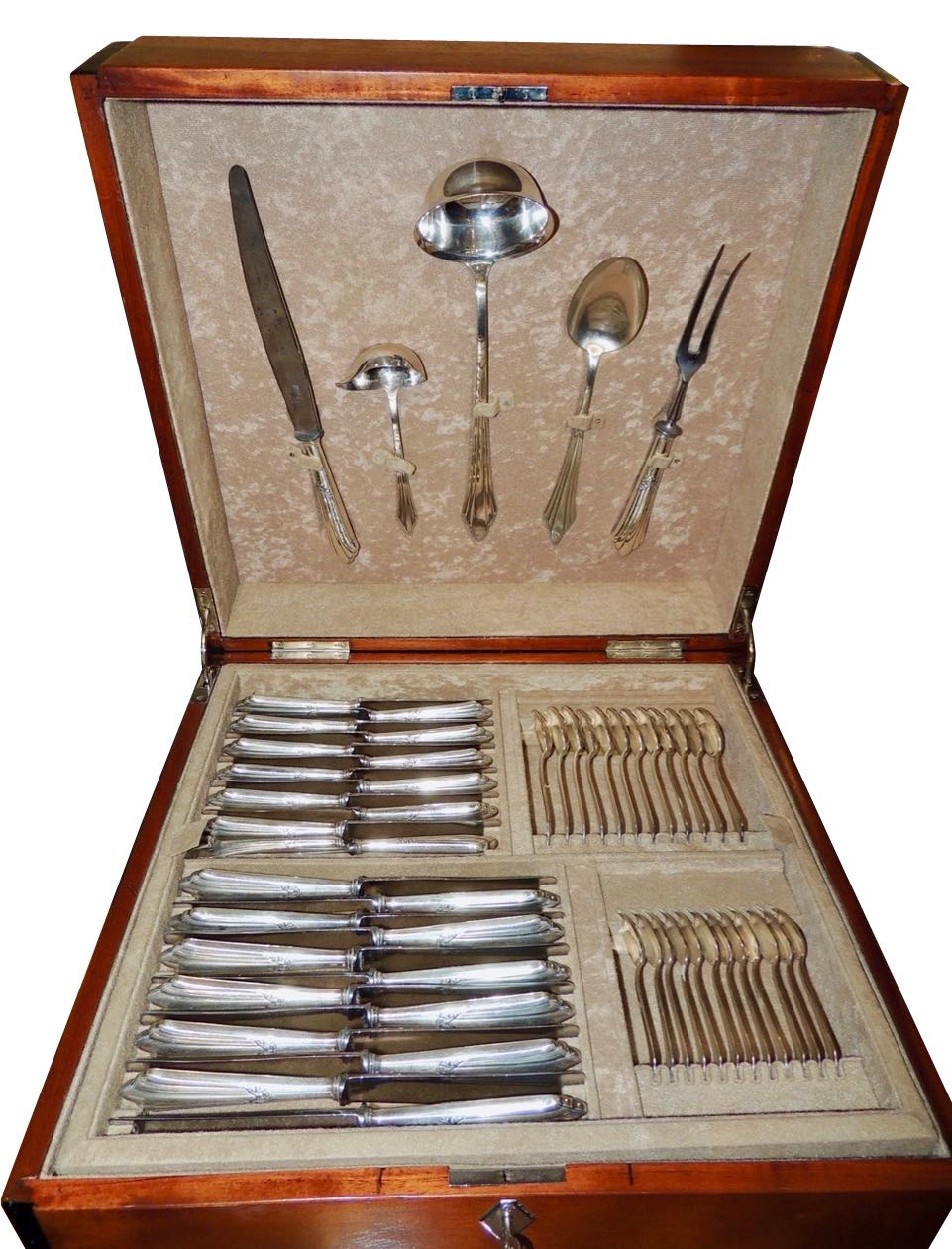The image shows an opened, dark brown wooden box containing an assortment of cutlery against a tan or beige background. The inside lid features an arrangement of silverware including a large bread knife, a big ladle, a small ladle, a soup spoon, and a pair of tongs. Below, the box is divided into four sections. The sections on the left hold horizontal rows of silver-handled cutlery, which appears to be a mix of spoons and knives. The sections on the right contain vertically aligned gold-colored cutlery, though it's unclear if these include spoons or knives. The interior seems to be lined with a velvet or cloth-like material, and the box features a silver latch on both the outside and the top.